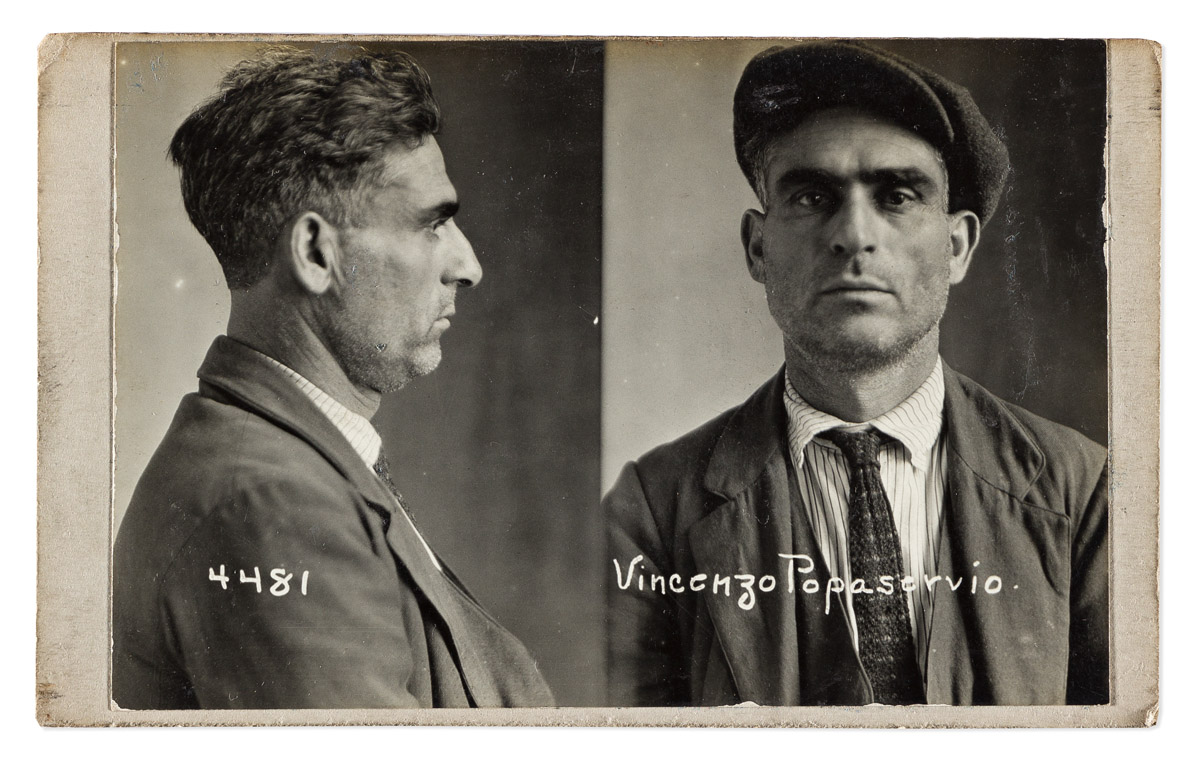The image is a black-and-white, early 20th-century mug shot of a Caucasian man named Vincenzo Pappaservio. It is divided into two photographs mounted on weathered, off-white cardstock, with the edges visibly aged and worn. The left-hand photograph shows the man's right profile, featuring his short brown hair, stubble, bushy eyebrows, and a prominent, slightly crooked nose. He is wearing a dark-colored suit, a white collared shirt with faint stripes, and a tie. Handwritten in white ink on this image are the numbers "4481" across his shoulder. The right-hand photograph depicts Vincenzo facing directly towards the camera, his facial expression serious and emotionless. He is now wearing a newsboy cap, his hair mostly hidden underneath. His attire remains the same, though his tie appears to be slightly askew and his jacket more disheveled. The name "Vincenzo Pappaservio" is handwritten in white ink across this photograph.